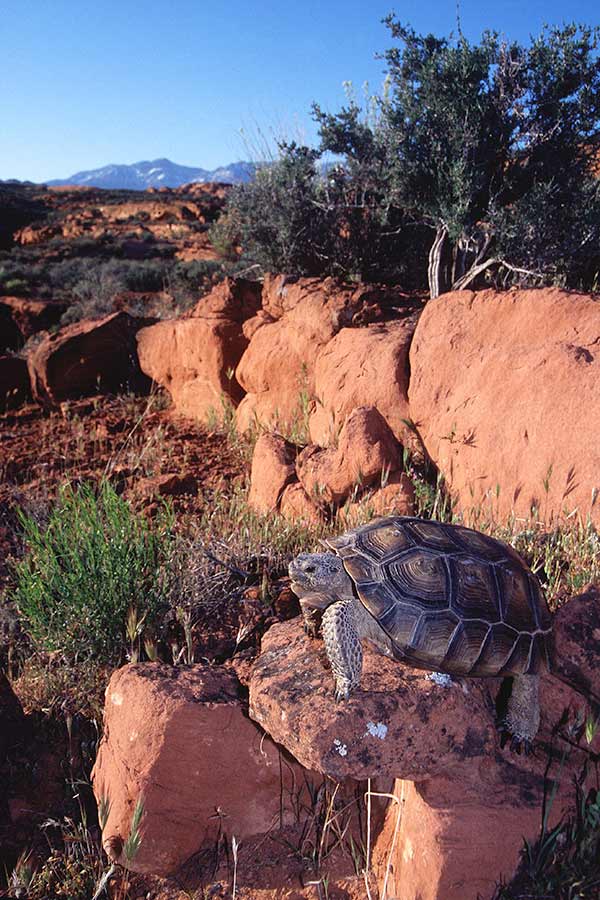This photograph captures an intriguing outdoor desert scene during daytime. Central to the image is a large tortoise perched atop a reddish-brown rock formation in the bottom right-hand corner. The tortoise, with its head out of its shell and its limbs firmly positioned, appears to be sunbathing. Its shell is predominantly brown, with black outlines and gray separations defining each section. Surrounding the tortoise, there is an array of green sagebrush and dried grass, typical of the arid terrain. To the left and behind the rocks, more greenery is evident, including additional sagebrush and possibly juniper bushes. Above the tortoise, a cliffside extends from the right, composed of large reddish-brown stone boulders adorned with sparse vegetation. In the background, the landscape stretches out to reveal distant mountain ranges beneath a clear, vivid blue sky, enhancing the rugged and serene desert atmosphere.